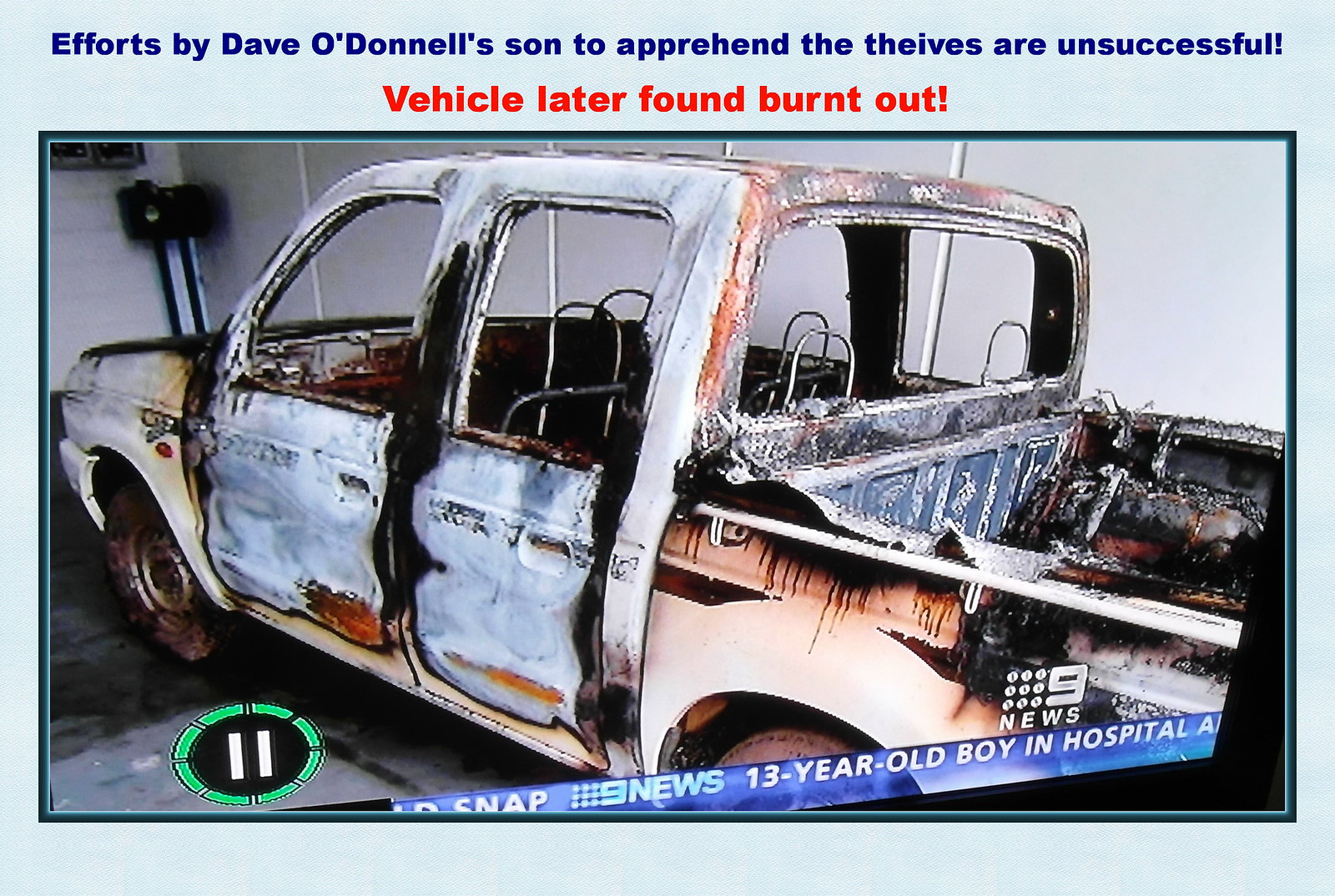This is a screenshot from a 9 News broadcast featuring an image of a completely totaled pickup truck that was both stolen and set on fire. The truck appears to have originally been white, but the intense fire burned through to the blue primer color and charred the interior and truck bed black. The photo includes a blue, matte border around it. At the top in blue text is the phrase, "Efforts by Dave O'Donnell's son to apprehend the thieves were unsuccessful," followed by red text stating, "Vehicle later found burnt out." The bottom right corner of the screenshot displays the 9 News logo, while a blue banner running across the bottom states, "9 News 13 year old boy in hospital." Additionally, a pause button icon is visible in the lower left corner, suggesting the image was captured from a paused video segment on a TV or computer screen.